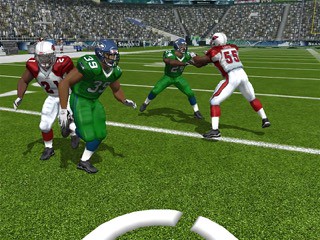A screenshot from an American football computer game captures a mid-action scene on the green gridiron field. The angle suggests a sideline view, showcasing part of the field extending into the distance. At the top of the image, spectators are visible in the stands, adding to the immersive gaming experience. The focus is on four football players on the field: 

On the left, a player in a green uniform and blue helmet is running towards the right. Close behind him, another player in a red and white uniform, wearing a white helmet, is in pursuit. In the upper right, another player in a green uniform is poised with legs spread wide and hands out, likely attempting to block or tackle. Facing this player is an opponent, dressed in a red and white uniform, who appears to be engaged and ready to counter the move.